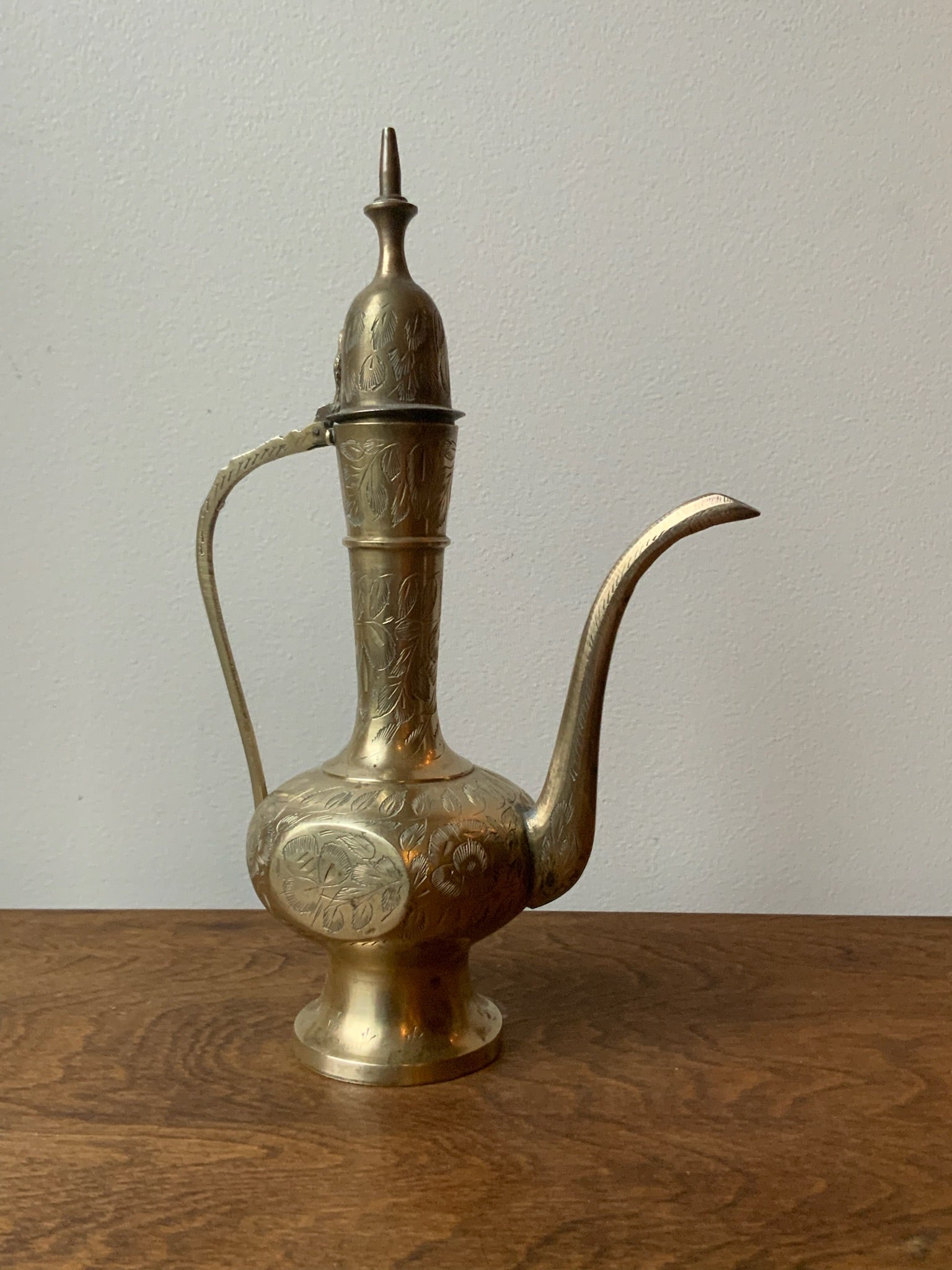This close-up photograph features an antique Middle Eastern brass kettle, reminiscent of a hookah or a vintage tea kettle, showcased as a standalone object. The kettle is positioned atop a naturally grained oak surface, either a table or a bookshelf, set against a plain white painted wall. The brass vessel exhibits an intricate design with etched leaf and floral motifs adorning its entire exterior. A long, thin, and delicately curved spout extends upward from the right side of its round base, while a prominent curved handle rises from the left side, arching over to meet a hinged lid at the top. The kettle's patina and ornate detailing suggest a historic and possibly utilitarian object, evoking imagery of classic genie lamps.